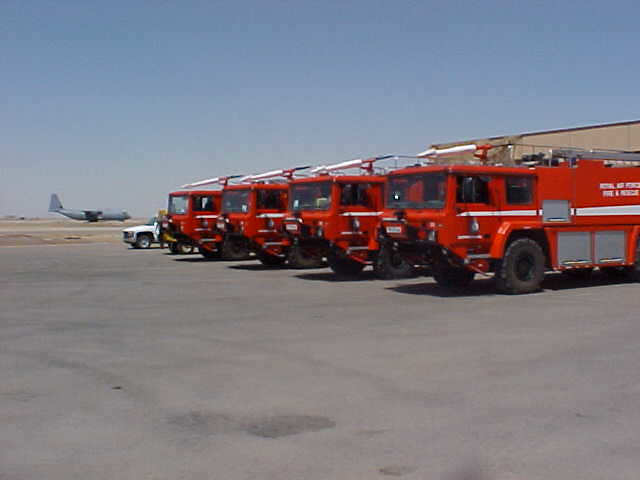This photograph captures a fleet of four identical red fire trucks, each adorned with metal ladders on top, large glass windows in the cab, and side mirrors. Despite some light stains and water markings on the smooth paved cement surface of the expansive parking lot, the scene exudes orderliness. The fire trucks, featuring black rubber tires and white stripes through the middle, are aligned uniformly, pointing outward into the lot. In front of them stands the top edge of a brown shed or garage building, while the front end of a white car peeks out from behind the last truck. The sky above is a deep, clear blue, though a slight layer of fog or dirt can be seen at the horizon. In the distant background, beyond a field that looks like a runway, sits a small gray airplane, its status—either parked or preparing for takeoff—uncertain. The fire trucks bear some gray panels that likely house tools or equipment, and the first truck's side features partial white text, with "fire and rescue" discernible. This meticulously captured scene suggests an older photograph, potentially taken in a desert-like setting.